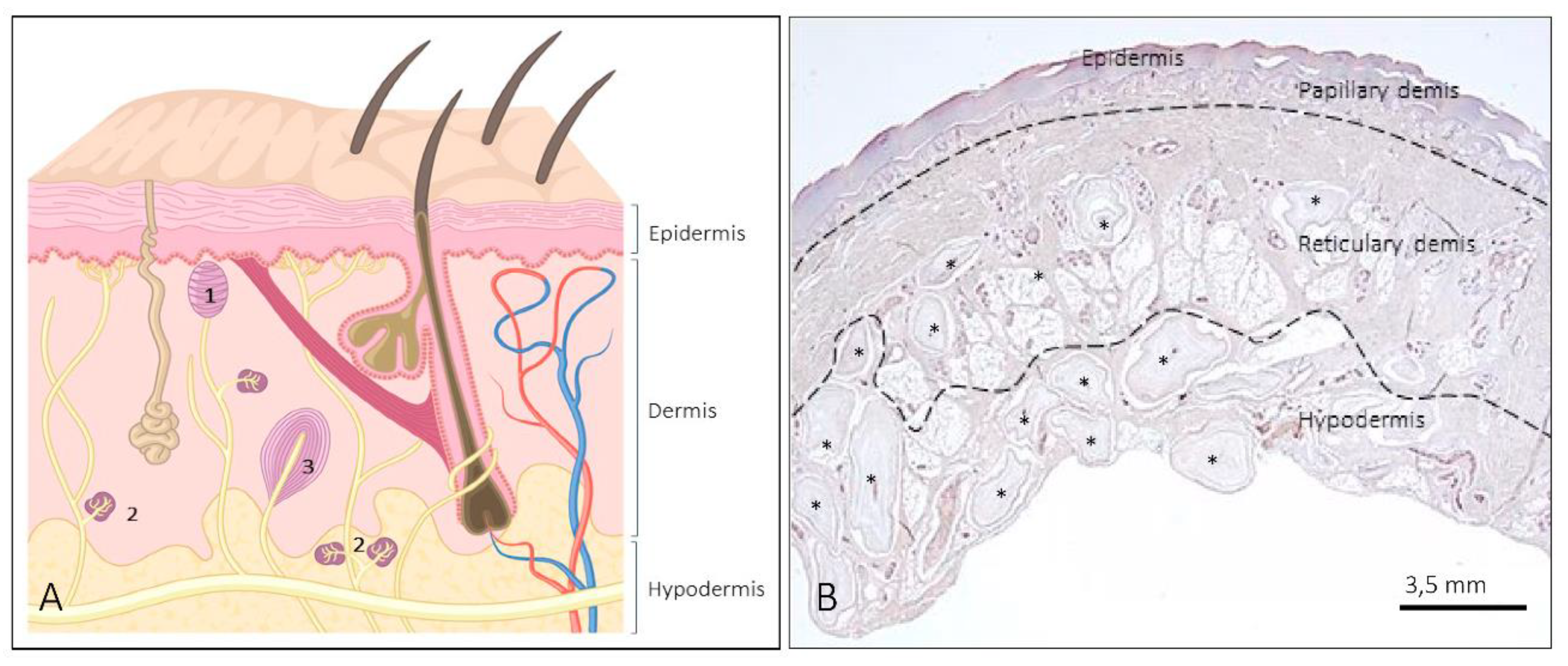This image consists of two side-by-side diagrams on a white background. 

The left diagram, labeled "A," is a colored, cutaway section of the skin, illustrating its surface layer and underlying structures. This detailed representation includes four whiskers protruding from the top, with hair follicles extending deep into the sublayers, shown as darker brown recesses. The skin layers are labeled as the epidermis at the surface, the dermis in the central region, and the hypodermis in the deepest part. Additional features include scattered numbered pink objects, likely indicating various skin components, and squiggly pink and blue lines on the right side, representing blood vessels or nerves.

The right diagram, labeled "B," is a grayscale scientific rendering, more technical in nature, showing a curved, arched surface near the top. This figure includes a legend with a 3.5 millimeter scale. The diagram's central squiggly, uneven rippling dotted line divides the epidermis from the deeper layers. Underneath these lines, various circular structures with black centers are visible. The diagram labels the layers as the epidermis, papillary dermis, reticular dermis, and hypodermis, providing a detailed comparison of tissue thickness and structural relationships.